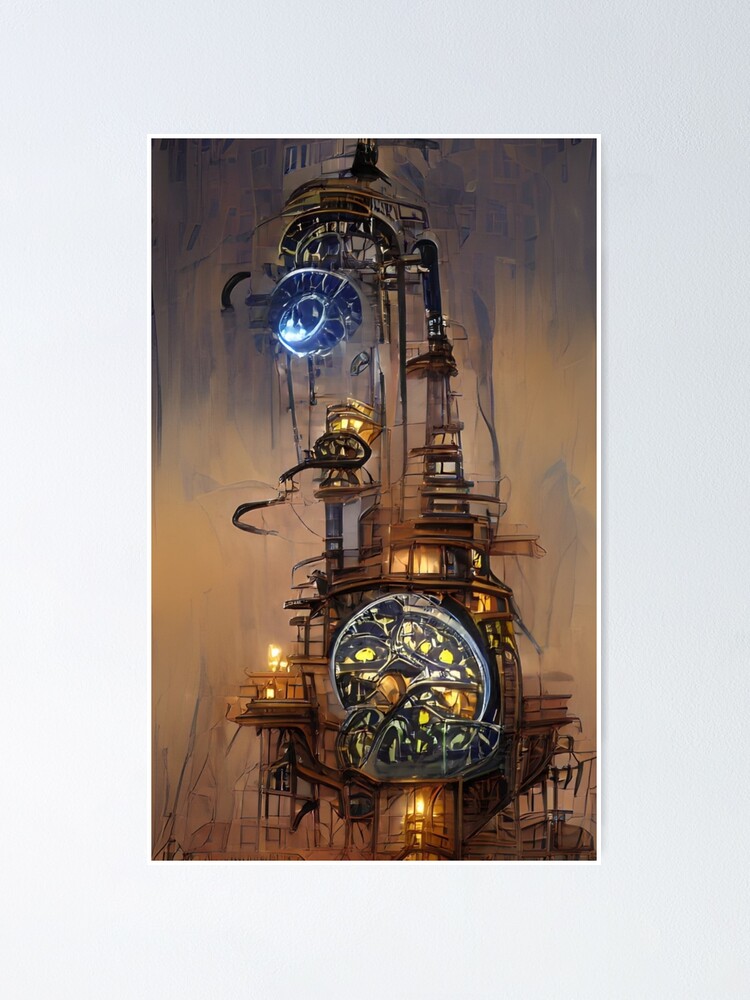The image is a tall, rectangular painting resembling a smartphone screen, with a thin white border against a light gray background. It depicts an abstract, steampunk-inspired structure that appears both fantastical and mechanical. The tower-like design is adorned with spires and towers, interspersed with large, bulbous glass elements that might serve as rooms or observation areas. The overall color palette includes prominent gold, brown, and bronze hues, contributing to its steampunk aesthetic. At the bottom of the structure is a glass-like orb with glowing yellow elements, evoking a sense of clockwork intricacy. Higher up, a smaller arch cradles a blue, electrically illuminated orb, adding to the surreal, almost Jules Verne-like atmosphere. Portions of the structure display features reminiscent of oil platforms, with illuminated windows and hints of flames. The nebulous and expressionistic style, potentially AI-generated, lends the painting an ethereal quality, making some details appear physically improbable.